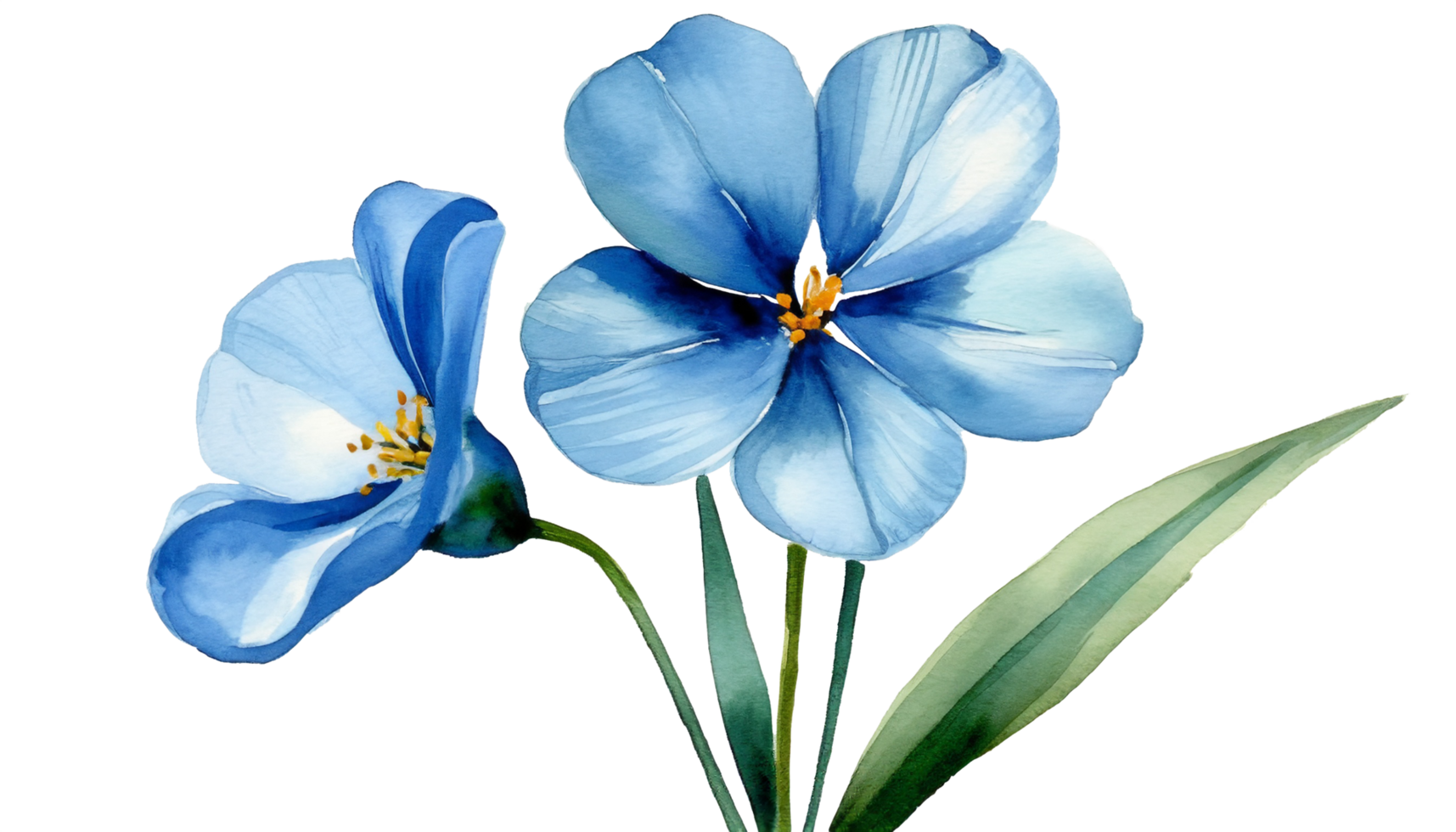This exquisite watercolor painting features a central flower with five delicate blue petals, beautifully detailed with a gradient that transitions from a deep, dark blue near the center pistil to a softer, light blue wash at the edges. The pistil itself is strikingly orange, adding a vibrant contrast. To the left of the main flower, another bloom emerges, depicted from a side view, gently extending out of the frame to the left. The flowers are accompanied by long, slender leaves, meticulously shaded in varying hues of green, adding depth and realism to the illustration. The composition is set against a pristine white background, which accentuates the bright and lively tones of blue, yellow, and green, allowing the colors to truly pop. This artwork captures the simple yet captivating beauty of the blossoms with a vivid and enchanting palette.